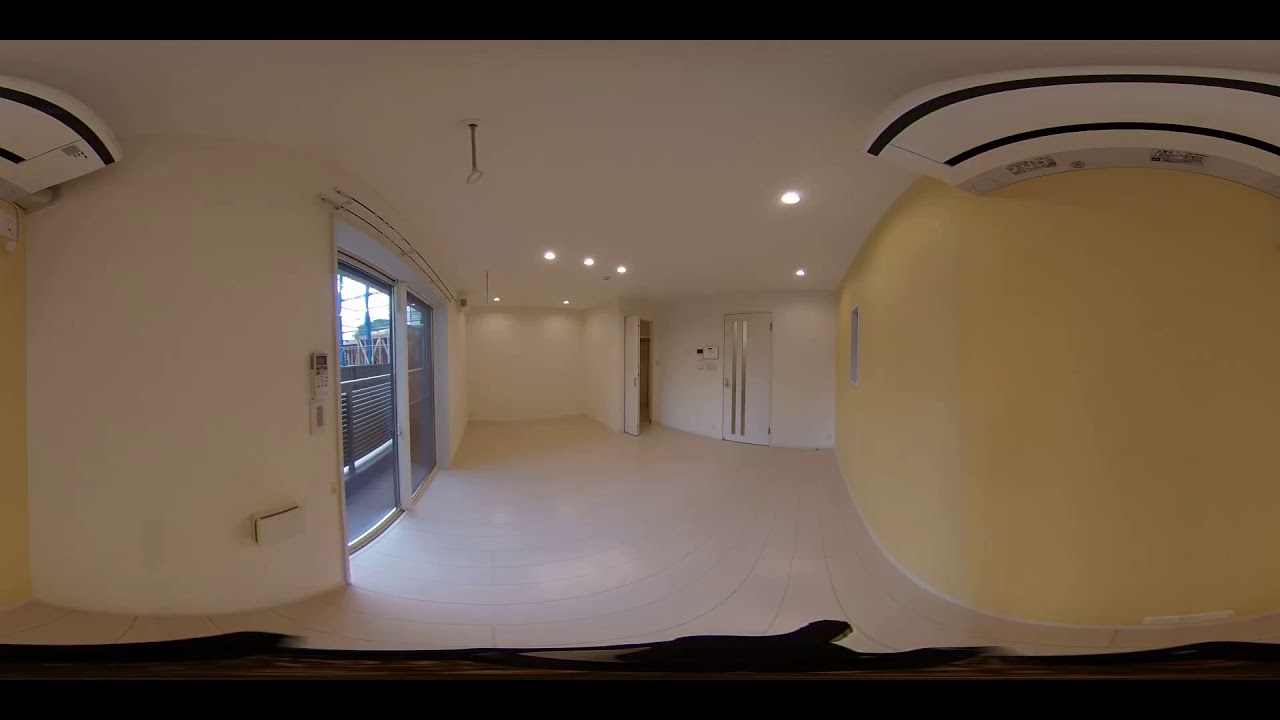This photograph, captured with an unusual lens that distorts the perspective and bends the walls, provides a dynamic view of a modern, likely unoccupied entrance area. The image is horizontally rectangular, showcasing a predominantly white or off-white interior. The floor and walls are uniformly light-colored, enhancing the stark, clean aesthetic. Distinctive black borders frame the top and bottom of the image. 

On the left side, a glass entrance suggests an office building, possibly opening onto a balcony as indicated by a adjacent slider. Before this entrance, a corridor curves leftward, adding a sense of depth. On the right, another corridor similarly extends out of frame. Directly ahead, a closed door punctuates the scene, possibly leading to an office or another room. The ceiling is dotted with round lights, illuminating the area evenly. The setting is devoid of any furnishings, emphasizing its vacant, pristine state.